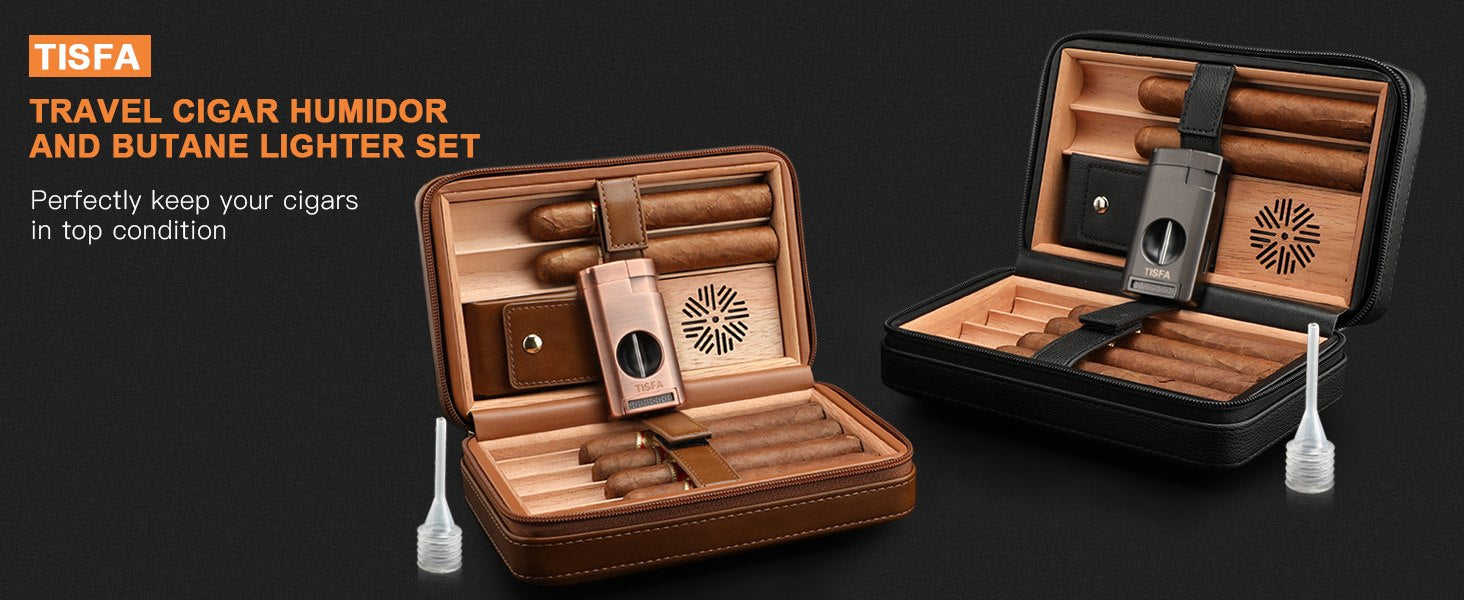This horizontally aligned rectangular image features a product advertisement with a solid black background. Prominently placed in the upper left corner, the text "T-I-S-F-A" appears in white against an orange background, followed by "TRAVEL CIGAR HUMIDOR AND BUTANE LIGHTER SET" in all caps, brown lettering. Underneath, in smaller white letters, is the slogan "Perfectly keep your cigars in top condition."

The center of the image displays two open cigar cases facing the viewer. On the left, the brown leather case has two cigars secured at the top and a small brown compartment resembling a cell phone holder underneath, along with five cigars lying flat at the bottom. The right side features a nearly identical black leather case with two cigars at the top and four or five cigars lying flat at the bottom, along with a black compartment. Each case also includes a lighter—copper-colored for the brown case and gray for the black one. Additionally, a clear cap-like item is visible next to the cases. Both cases and their contents are meticulously arranged, emphasizing their functionality and sophisticated design.